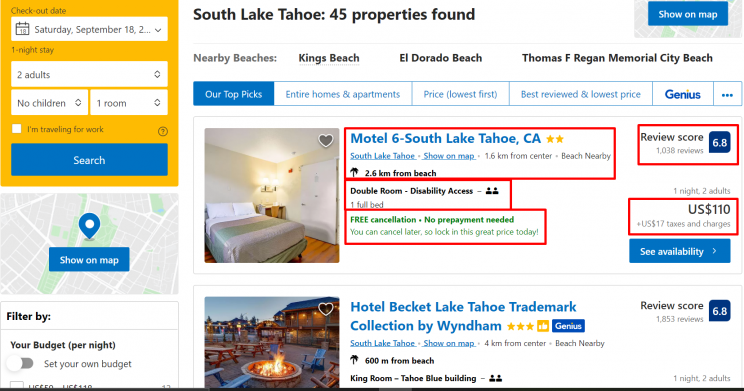An online hotel booking interface is displayed in this image, showcasing search results for accommodations in South Lake Tahoe. At the top of the screen, a banner announces "South Lake Tahoe, 45 properties found." On the left side, search criteria are clearly defined: the checkout date is set for Saturday, September 8th, with a one-night stay for two adults, no children, and one room. A prominent blue "Search" button is visible below these details. 

Under the search options, a map view can be toggled with another blue button labeled "Show on map." 

On the right side, search results begin with two highlighted options. The first listing is Motel 6, South Lake Tahoe, CA, rated with two stars. Important details are emphasized with red borders: a review score of 6.8 based on 1,038 reviews, pricing of US $110 for the night with an additional US $17 for taxes and charges. The listing specifies a double room with disability access, one full bed, free cancellation, and no prepayment required, advising, “You can cancel later, so lock in this great price today.” A thumbnail image of the motel room, featuring a bed and some lights, is included below the text.

The second listing features Hotel Beckett, Lake Tahoe Trademark Collection by Wyndham, boasting three stars. The accompanying image showcases an inviting exterior with numerous chairs arranged around a central campfire-like feature. 

Each listing provides essential information and visual snapshots to aid in making an informed booking decision.